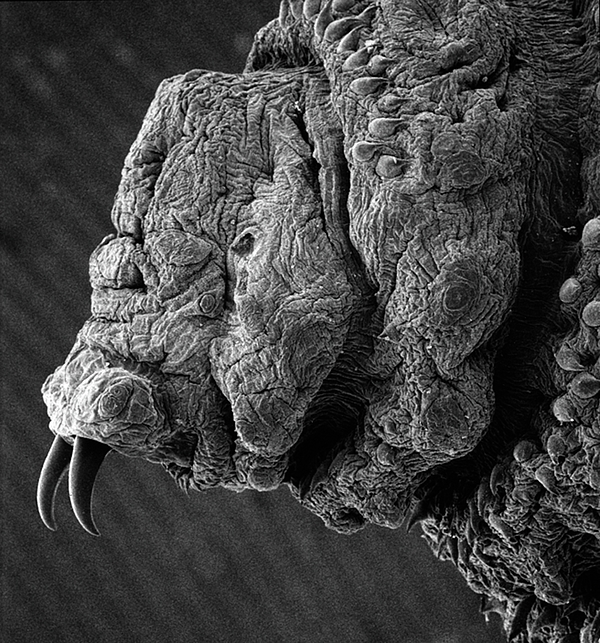The black-and-white image depicts a grotesque and unsettling creature, seemingly a blend of various animals and perhaps even an artistic carving. The creature's face appears deformed, melted, or molted, giving it an unnatural and eerie appearance. Its crinkly, grayish skin resembles that of an elephant, while the top of its head bears spikes reminiscent of a Triceratops dinosaur. Prominent features include two large, sharp black tusks or fangs protruding from its mouth. The creature's neck is adorned with small, round bumps, adding to its bizarre and menacing presence. The overall impression is that of a demented walrus or a dragon, with some parts looking like unfinished carved wood. The image conjures a sense of unease, as the creature appears menacing and potentially harmful.